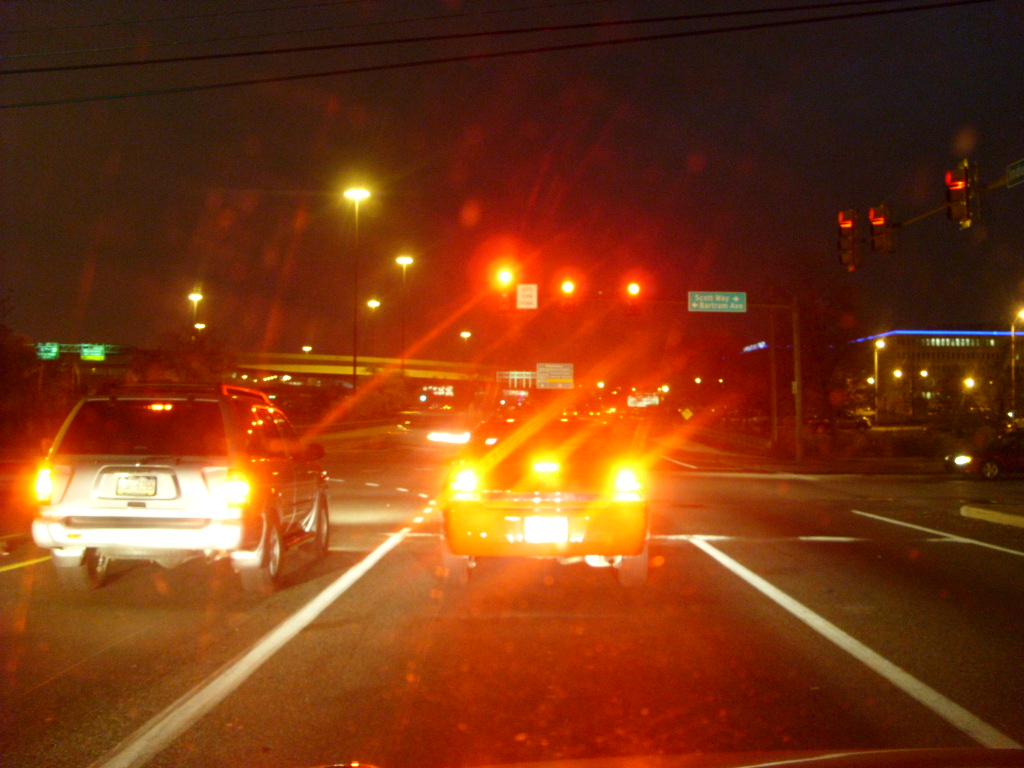This nighttime photograph, taken from inside a car waiting at a red light in the middle lane, showcases a city street illuminated by bright, glowing traffic lights. Directly in front of the car is a small four-door sedan with its intense brake lights visible. To the left of the sedan is a grey SUV. Adding to the urban ambiance, a green street sign is affixed to the same pole holding up the traffic signals. In the background, a large building to the right is adorned with a striking blue LED light strip running under its roof, while an overpass can be seen towards the middle of the image and to the left. The scene has a slight blur, emphasizing the glow of various city lights and headlights that pierce through the darkness.